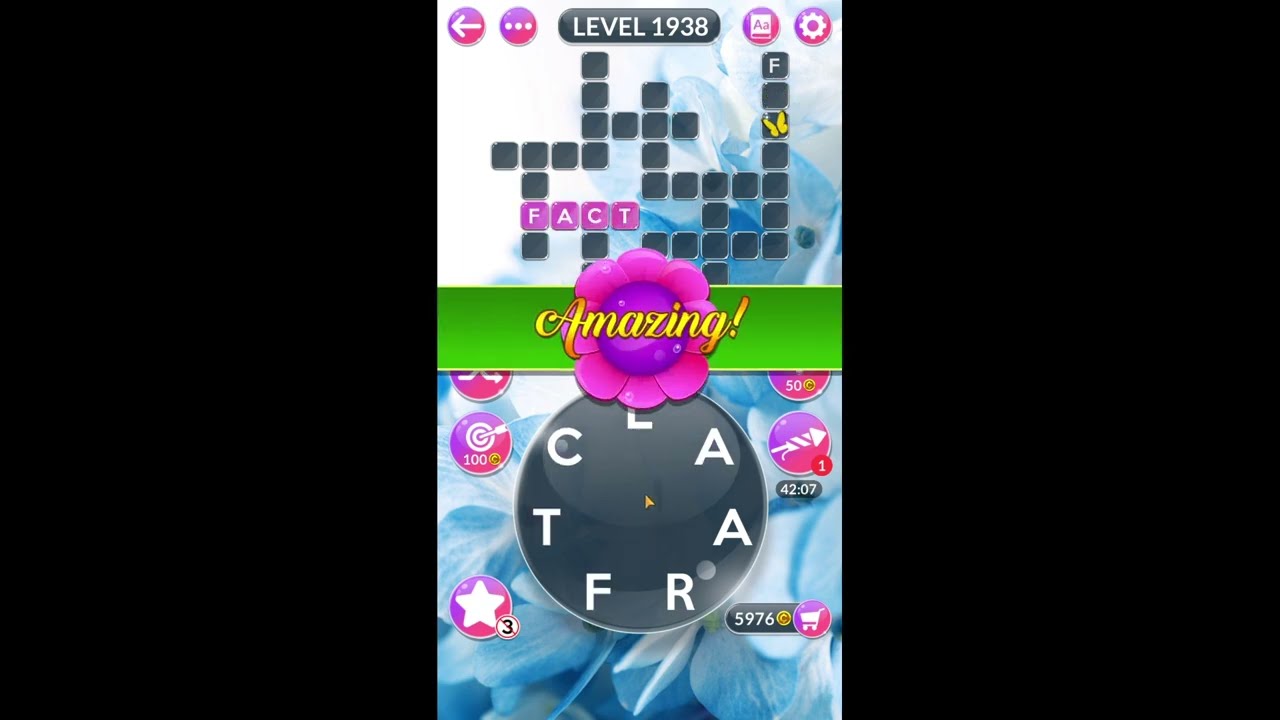This image is a screenshot of a smartphone game that resembles Scrabble or a crossword puzzle. The main screen is visible, flanked by blacked-out sections on the left and right, accentuating the central gameplay area. At the top of the image, positioned within a black oval, is the text "Level 1938" in white. To the left of this label, there are two red circular icons; one featuring a left-facing arrow and the other, three green dots. On the right, two additional red icons include the letters "AA" in one and a settings gear in the other.

Just below this top section, we enter the game itself, which displays a black crossword grid with most tiles obscured. The visible word "FACT" is displayed in white on pink tiles toward the lower half of the grid. In the center of the screen, a green banner adorned with purple and pink flowers carries the word "Amazing!" in yellow cursive text, adding a celebratory touch. 

Beneath this floral banner lies a large black circle, assembles with the letters L-A-A-R-F-T-C arranged in a clockwise pattern. The circle likely functions as a letter wheel for the game. Additional icons around this circle include arrows and a bullseye, and at the very bottom right corner, there's a small basket icon accompanied by the numbers 5, 9, 7, 6 and a yellow coin.